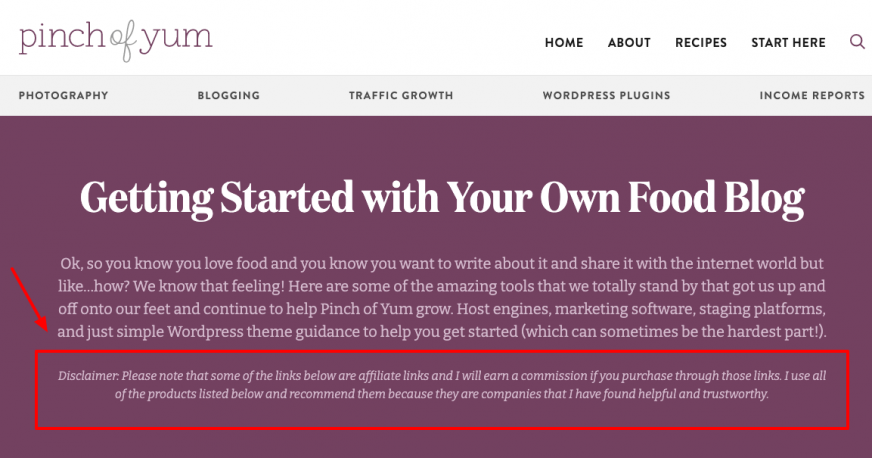The top section of the page features the "Pinch of Yum" logo, elegantly designed with "Pinch" in purple, "of" in grey, and "Yum" in purple again, on a white background. Above this logo, the navigation bar, in black, displays various tabs including Home, About, Recipes, and Start Here with a purple highlight, as well as a search icon represented by a magnifying glass.

Beneath this border is a secondary grey navigation strip, listing more tabs in dark grey: Photography, Blogging, Traffic, Growth, WordPress, Plugins, and Income Reports. The background of the page has a rich plum color, giving it a warm and inviting tone.

Prominently displayed in bold white text and large font are the words "Get Started with Your Own Food Blog." Below, in smaller, non-bold white text, it reads: "Okay, so you know you love food and you know you want to write about it and share it with the internet world, but like... how? We know that feeling! Here's some of the amazing tools that we totally stand by that got us up and off onto our feet and continue to help Pinch of Yum grow: hosting engines, marketing software, staging platforms, and just simple WordPress theme guidance to help you get started, which can sometimes be the hardest part."

On the left-hand side of the page, a red arrow points to a box outlined in red. At the bottom of this box, a white disclaimer reads: "Please note that some of the links below are affiliate links and I will earn a commission if you purchase through those links. I use all of the products listed below and recommend them because they are companies that I have found helpful and trustworthy."